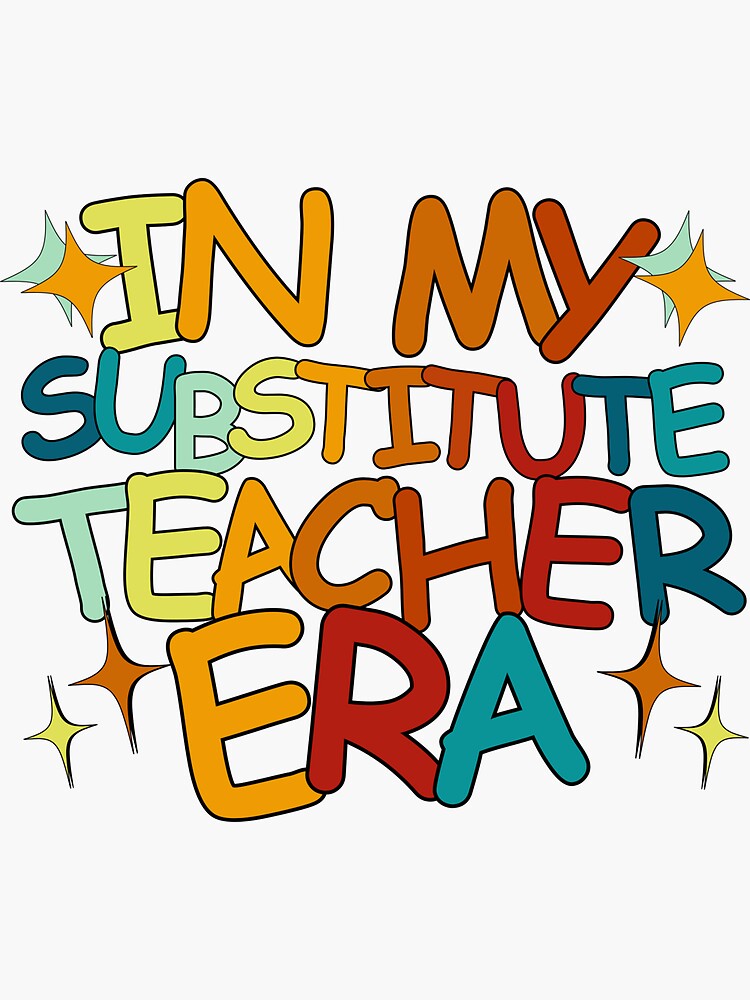The image displays a vibrant poster with the phrase "In My Substitute Teacher Era" in varied, playful uppercase letters. Each letter is uniquely colored in a palette of lime green, orange, burnt orange, red, teal, and light blue, arranged in an irregular and overlapping fashion, with some tilted at various angles. The background is off-white with a subtle bluish tinge. Surrounding the text are four-pointed stars in colors of teal, orange, and yellow. Specifically, there are two stars to the left of "in" and two stars to the right of "my". At the bottom of the image, two stars appear to the left and right of "era," colored in yellow and orange, respectively. The overall chaotic but charming design, with its blocky, black-bordered letters scattered 'messily' around the image, creates a lively visual likely intended for a promotional or artistic classroom piece.